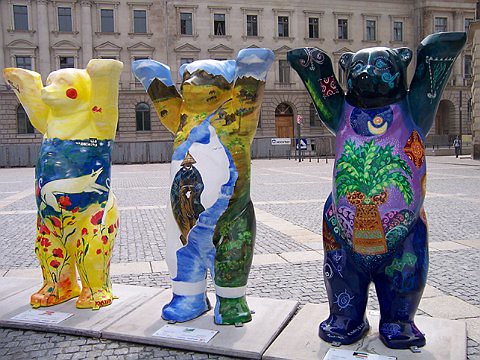In this detailed photograph of an outdoor scene, we see a tranquil town square dominated by a stately, three-storied European-style stone building in the background, accented with many rows of windows and enclosed by an iron fence. The foreground features a cobblestone walkway, upon which stand three vividly painted bear statues, each raising their arms upwards. The leftmost bear is adorned in yellow with blue accents and red feet, embellished with flower motifs. The middle bear showcases a scenic landscape painted in greens, blues, and yellows, depicting elements like trees and mountains. The rightmost bear, painted in purples and blues, boasts an artistic design with decorative flowers and a prominent moon on its chest. The scene captures a serene moment with no visible people, highlighting the vibrant artistry of the statues against the historic and architectural charm of the surroundings.